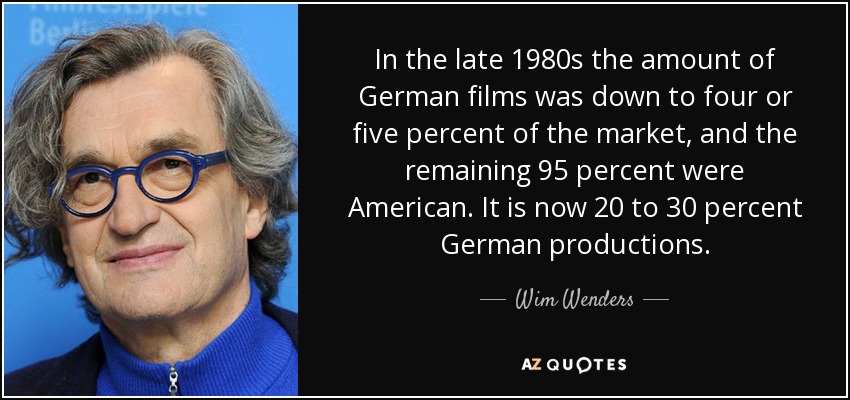The image features a headshot of an older man with longish gray, wavy hair parted on the side, extending past his shoulders. He is wearing round, modern-looking blue glasses that complement his dark royal blue zip-up turtleneck sweater. Over the turtleneck, he dons a black suit jacket. Behind him is a blue backdrop with some writing, although it is not legible. To the right of the man's image, there is a black background with white text stating a quote: "In the late 1980s the amount of German films was down to 4 or 5% of the market, and the remaining 95% were American. It is now 20 to 30% German productions." The quote is attributed to Wim Wenders, as indicated by the text "Wim Wenders AZ quotes."